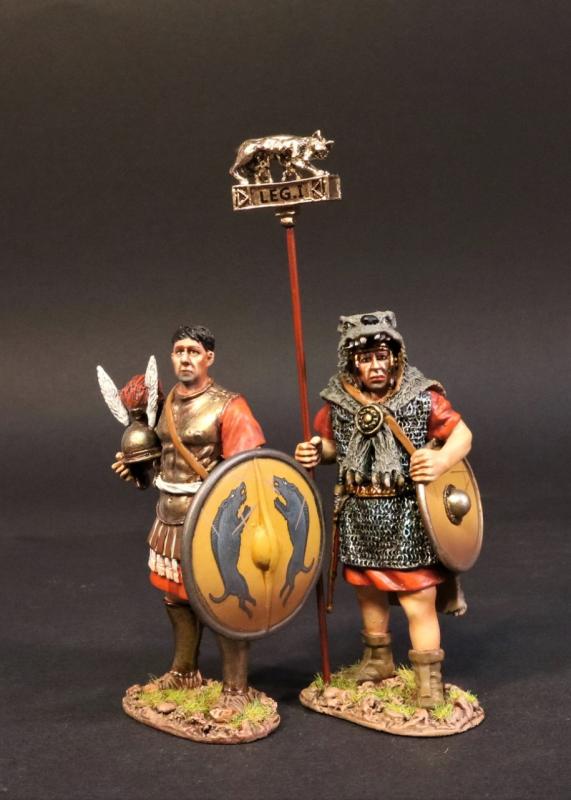This image showcases two intricately designed miniature figurines, each presented against a stark black background ideal for a detailed display. The first figurine depicts a Roman soldier adorned in period-accurate attire, featuring a gold or leather chest piece complemented by red sleeves and undergarments. He stands firmly on a tuft of grass, holding a yellow shield emblazoned with two wild boars in his left hand and a helmet with rabbit-ear-like protrusions and a red crest in his right. The second figurine represents a gladiator-like warrior, clad in chain mail over a red undergarment. This figure wields a round, minimally ornamented shield with a central gold stub in his left hand and a long pole topped with a brass or gold animal in his right. The two statuettes capture a moment of poised readiness, bridging historical influence with a hint of fantasy.